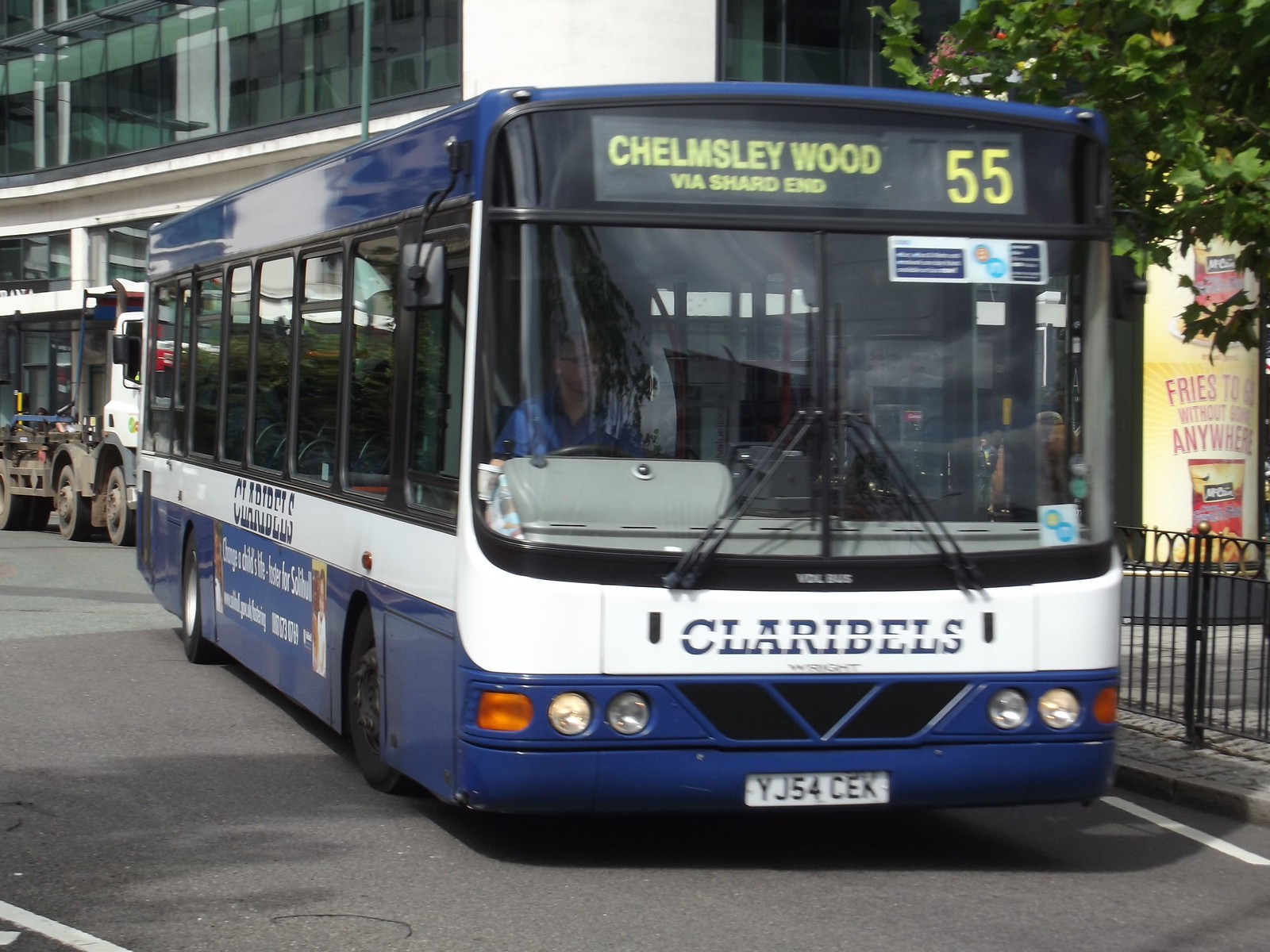The image depicts a predominantly dark blue city transit bus with a white stripe running along its middle section and wrapping around the front. The bus, which appears to be in England due to the driver being on the right side, features a green digital sign above the front windshield displaying the route information: "Chelmsley Wood via Shard End 55." Just below this digital sign, "Clarabelles" is written above the windshield, aligning with the bus's license plate number "YJ54CEK." 

Parked near a sidewalk by a building with numerous glass windows spanning its first two levels, the bus sits adjacent to a black metal fence. There is an advertisement behind the bus for McCain snacks that reads, "fries to go without going anywhere." Additionally, a holly tree is visible next to the bus on the upper right side of the image, and the hint of a possible tow truck behind the bus suggests it may have broken down. The side of the bus also displays the name "Clarabelles" and features large square windows.